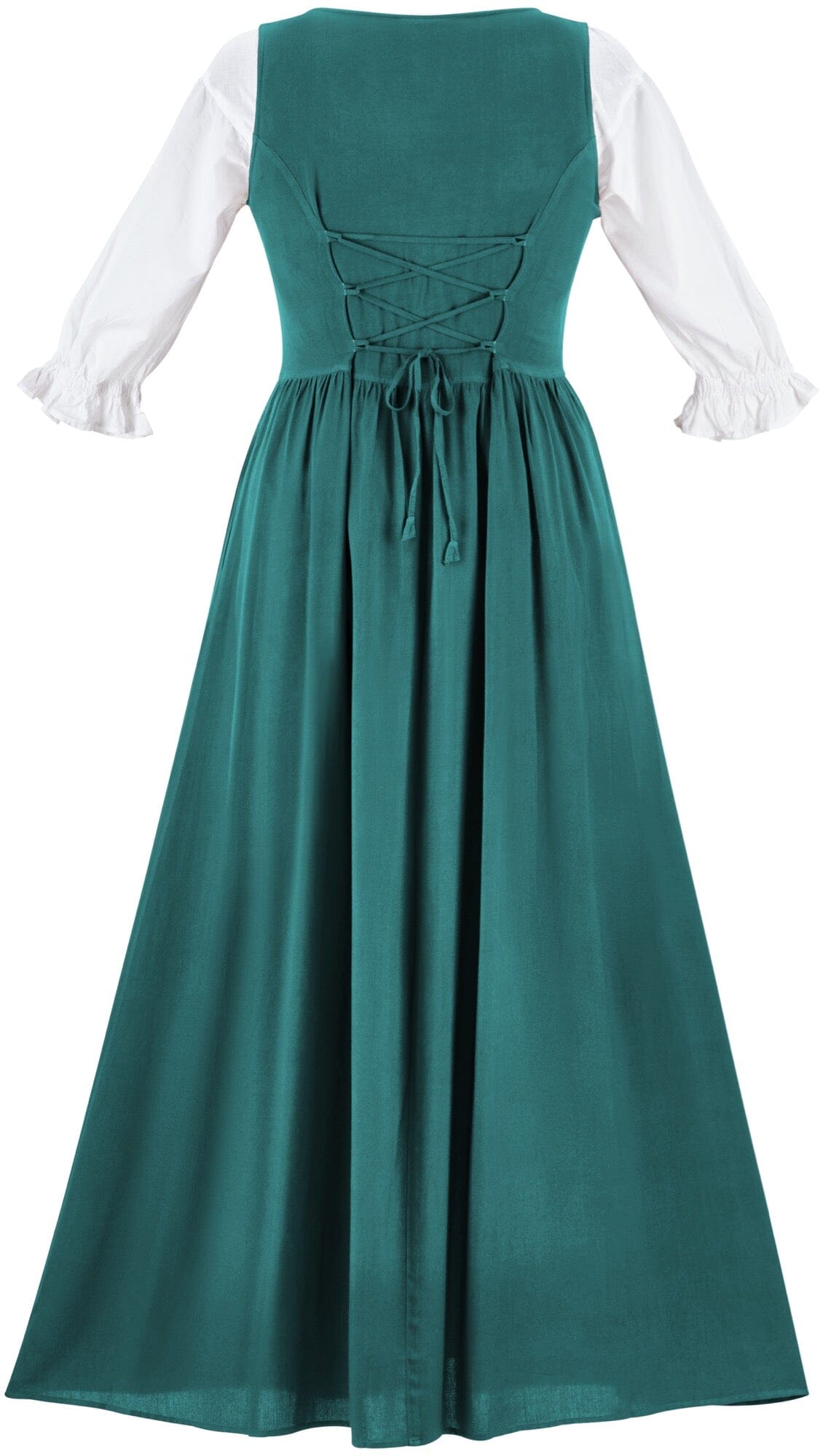This image features a detailed depiction of a historically-inspired, old-fashioned dress that appears reminiscent of the 1600s or 1700s. The dress is a long, ankle-length garment in a teal green color, made from what looks like a lightweight fabric, as the bottom of the dress shows some translucency, allowing the floor's reflection to be faintly visible through it. The dress has white long sleeves, which might either be part of the dress or a separate blouse underneath, adding to the garment's complexity. 

Displayed against a clean white background, the dress is shown from the back, highlighting its intricate lace-up design. The back of the dress features green ribbon laces that create two 'X' patterns near the upper back, then run straight across and tie off into a neat bow, with the ribbon tails cascading downwards past the midsection. This classic lacing detail, along with potential stays within the bodice, suggests a focus on historical accuracy in terms of dress construction and silhouette. Despite the dress's elaborate design, there is no mannequin or person wearing it, allowing full attention on the dress itself. The mixture of likely cotton or linen textures for the sleeves and a slightly shinier fabric for the teal portion creates a visually rich and authentically styled garment.